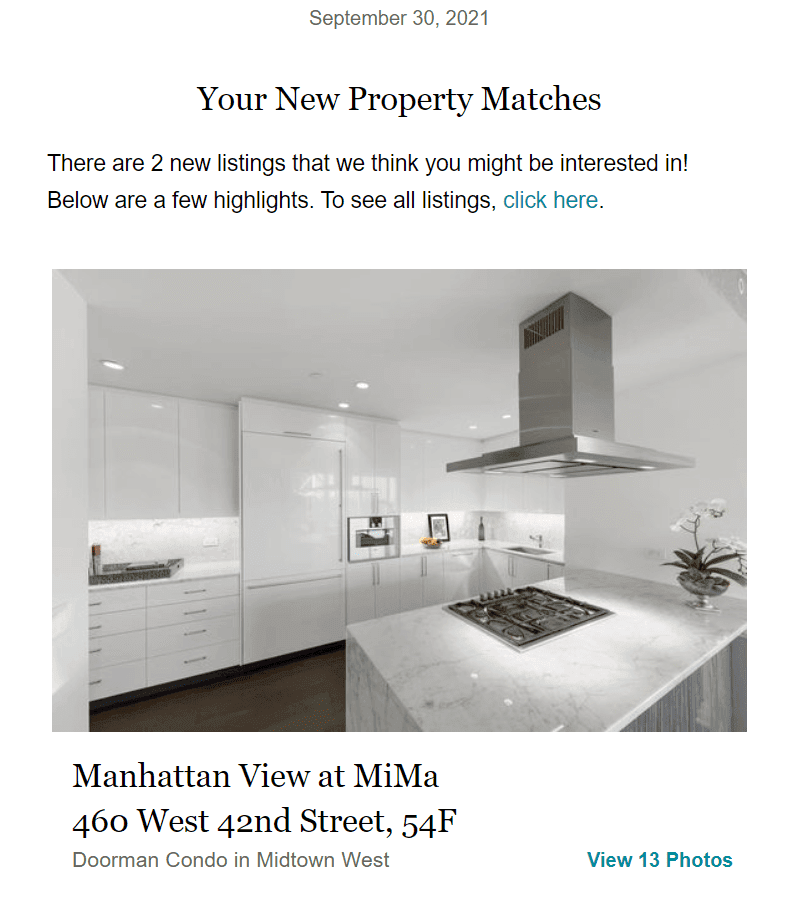This screenshot from a web page features a white background with black font text. At the top, centered, is the date "September 30th, 2021." Beneath the date, the heading reads "Your New Property Matches." Further down, in smaller font, a brief message states, "There are two new listings we think you might be interested in!" This is followed by "Below are a few highlights," and a hyperlink in blue text that says "To see all listings, click here."

Displayed below the text is a black and white photo of a very modern-looking kitchen. The kitchen features a sleek, redesigned cooktop surface and contemporary cabinetry. Under the photo, there is a headline that reads, "Manhattan View at MIMA," with the address "460 West 42nd Street, 54F" listed below. In gray font, the description reads, "Doorman Condo in Midtown West." On the right side, another hyperlink in blue font states, "View 13 Photos."